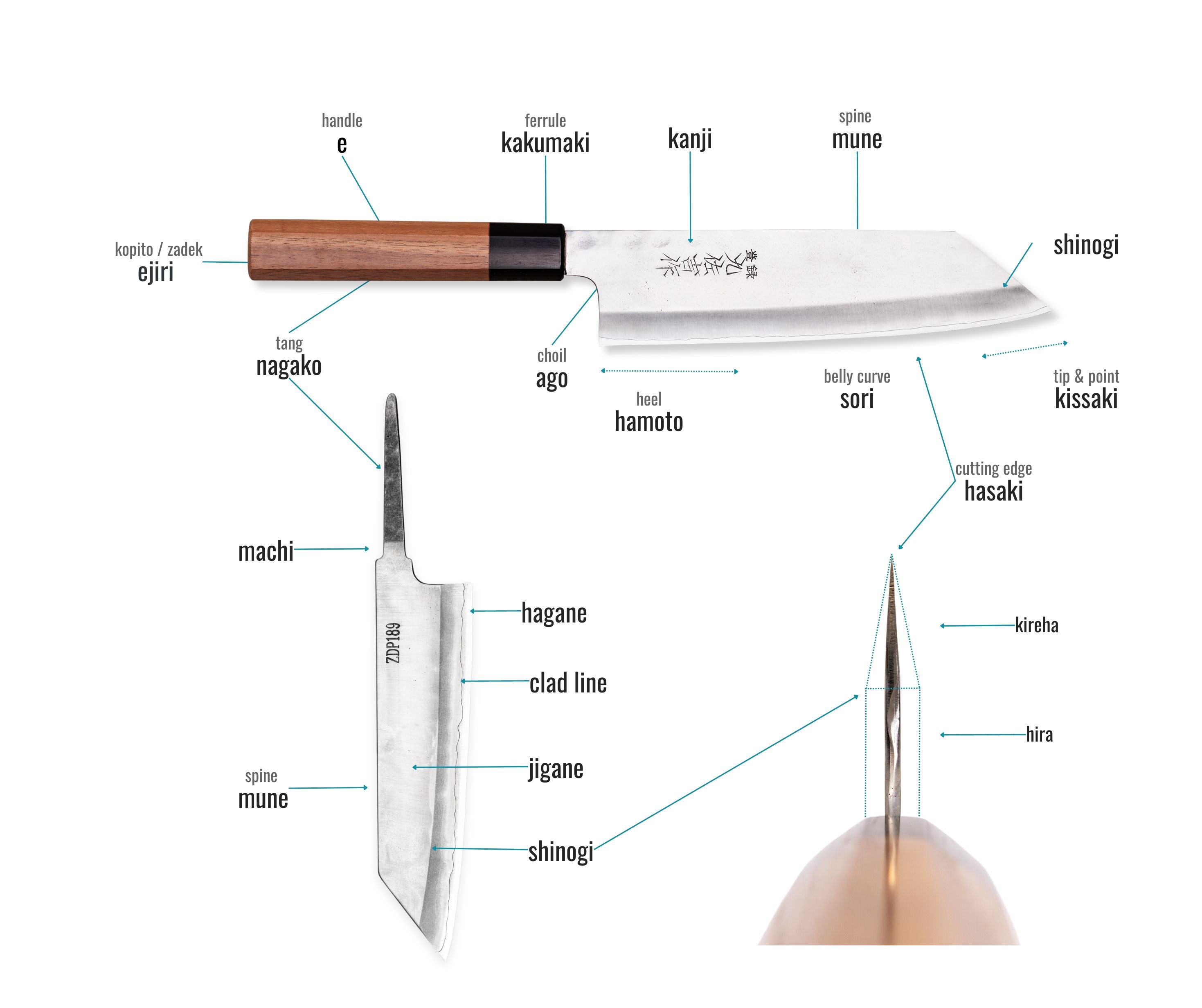The image is a detailed illustration series of a Japanese cutting knife, presented against a plain white background with no visible borders. The series includes three views of the knife, each meticulously labeled. 

At the top of the image, the knife is shown in a horizontal orientation, with the wooden handle to the left and the blade to the right. The brown handle is long and thin, adorned by a black ferrule labeled "Kakumaki," which separates it from the blade. Blue arrows point to various components with corresponding labels: Kopito Zadek Ejire (handle), Tang (part of the handle), Choil (the notch where the blade widens), Spine (Mune), Cutting Edge (Shinogi), Heel (Hamoto), Belly Curve (Rosori), and Tip/Point (Kisaki). The blade also features Kanji inscriptions.

Below this, there's a vertical drawing of the knife with the tip pointing downwards. The handle, labeled "Nagako," and the connection point "Machi" are detailed. The blade includes labels for Hagane (cutting edge material), Cladline, Jagane (cladding material), and Shinogi (cutting edge). The spine is again labeled "Mune."

In the bottom right corner, there's a close-up showing just the tip of the knife from a side view, highlighting the cutting edge labeled "Kuroha" and the flat part "Hira," with Shinogi also marked.

The labels are in black print, featuring both Japanese and English terms to describe each part of the knife meticulously.